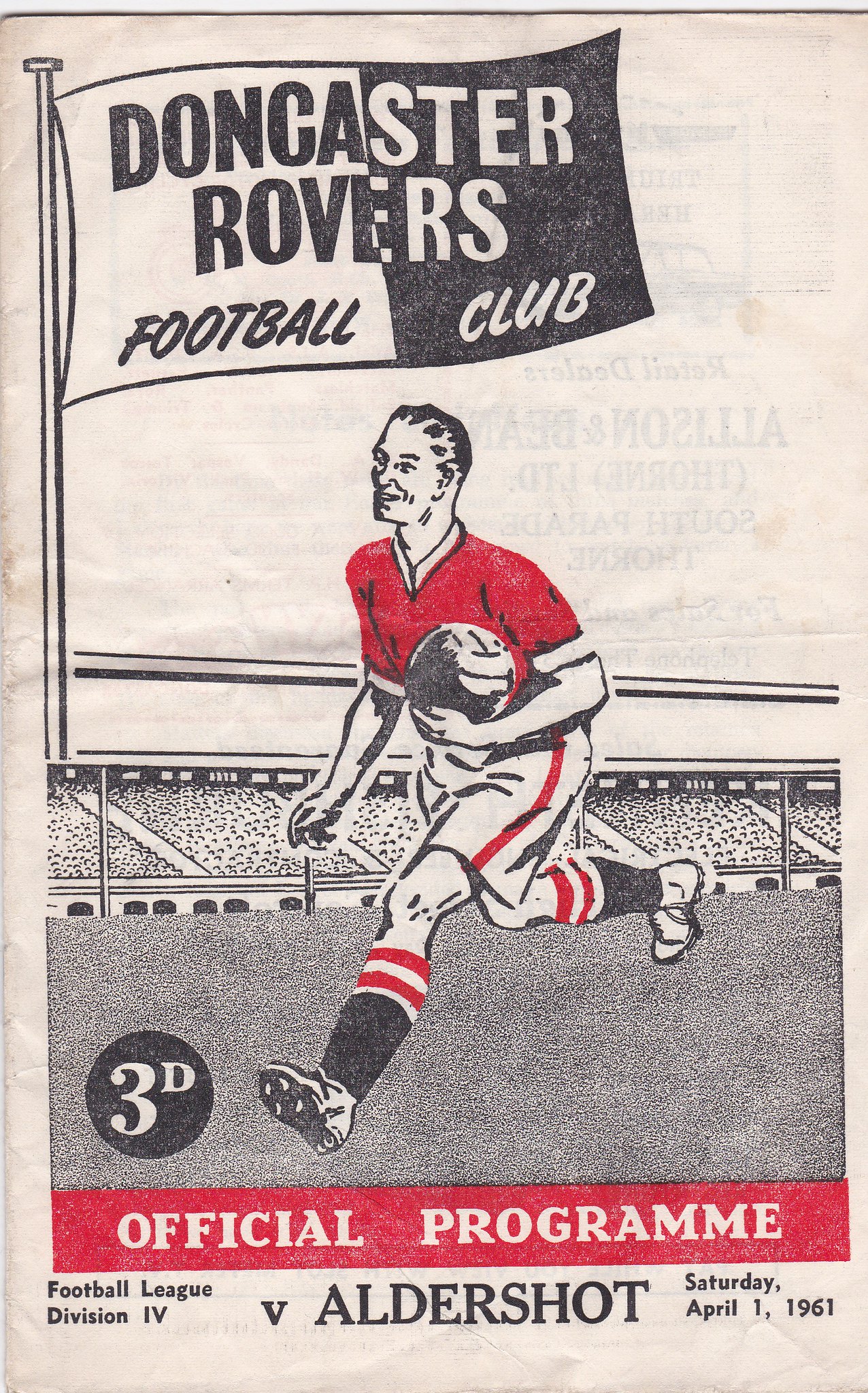This image depicts the front cover of a vintage soccer program on matte paper, showing signs of age with flaking and bends along the left-hand spine area. The background is white. Dominating the upper half of the cover is a large flagpole with a flag bearing the text "Doncaster Rovers Football Club." The flag is conspicuously divided into two halves: the left half is white with black text while the right half is black with white text. 

Below the flag is a detailed cartoon illustration of a soccer player. The player is shown running on a gray pitch and holding a soccer ball in his left hand. He is dressed in a red shirt, white shorts with a red stripe down the side, black knee-high socks with red and white stripes, and white cleats. Behind the player, there is a depiction of a stadium with stands filled with spectators.

Below the illustration, a red rectangular section contains the text "Official Program" in white letters. Further down, at the bottom of the cover, more black text on a white background details the event: "Football League Division IV v Aldershot, Saturday, April 1, 1961."